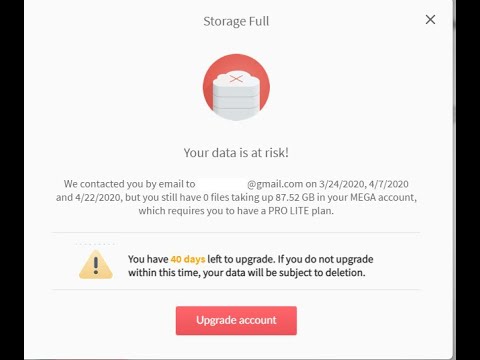**Caption:**

The image appears to be a notification from a web page, enclosed within a square interface. The right and left edges of the square are bordered by thick black lines, while the bottom edge has a very thin black line, and the top edge has no border but features a slightly grayer shade of white than the rest of the page.

At the top, the notification headline reads "Storage Full" with both 'S' and 'F' capitalized and a double space following it. There is a red circle partially visible, obstructed by an icon resembling three stacked tablets or pills with a red X over it. Below the icon, a warning message states "Your data is at risk!" with an exclamation mark and another double space.

The text explains that the recipient was contacted via email at a Gmail address on three dates: 3-24-2020, 4-7-2020, and 4-22-2020. Despite these notifications, the recipient still has zero files occupying 87.52 GB in their MEGA account, which necessitates a Pro-Lite plan.

Accompanying the warning is a caution logo. The notification informs the user they have 40 days left, highlighted in yellow, to upgrade. If the user fails to upgrade within this period, their data will be subject to deletion. At the bottom of the notification, there is a red rectangular button with white text that reads "Upgrade Account."